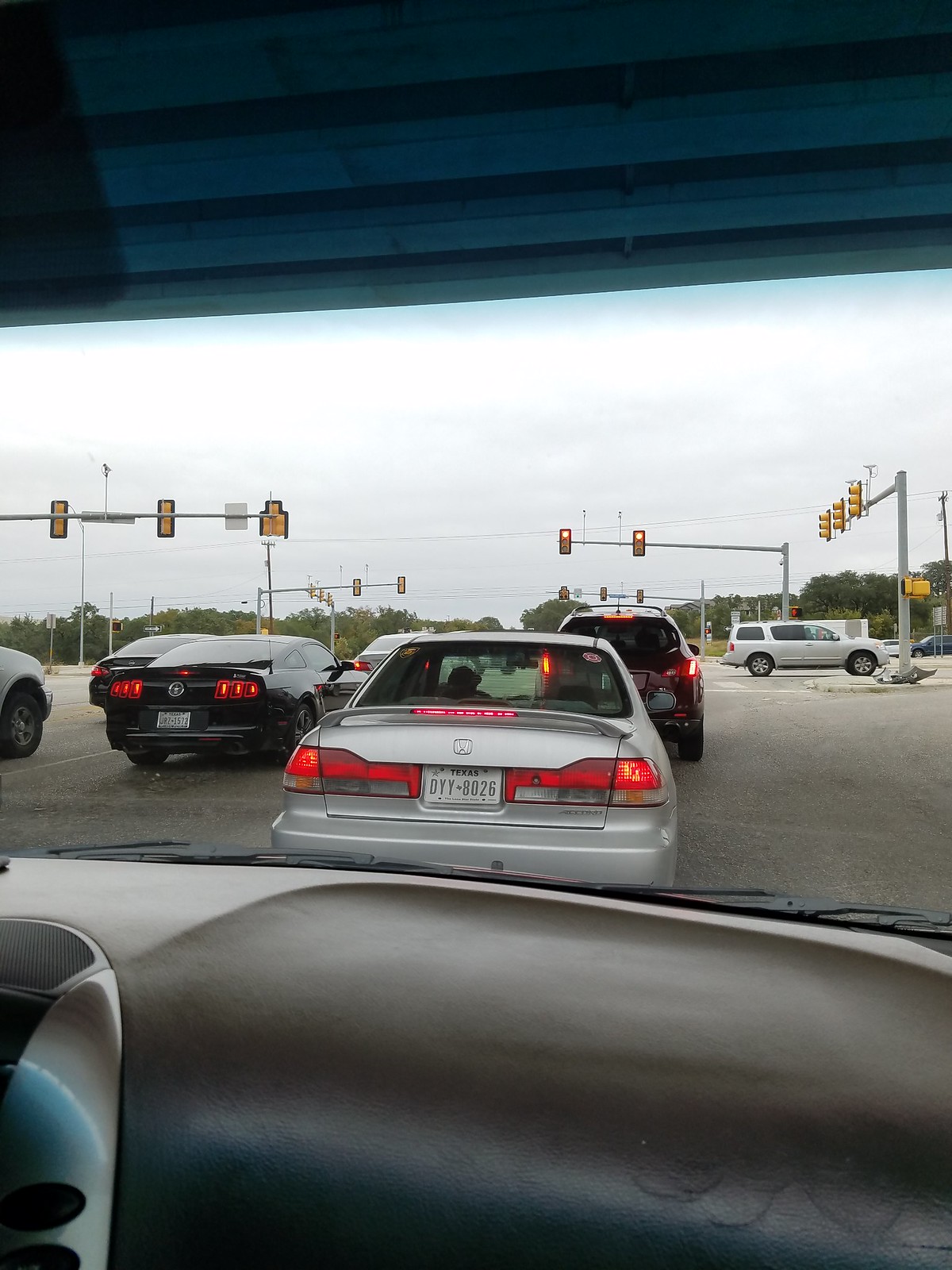The image depicts a moment of orderly traffic at a stoplight on a busy roadway. Positioned from the perspective of a vehicle's dashboard, which is dark gray and features black windshield wipers, the scene ahead includes a line of halted cars. Directly in front of the camera is a gray car, followed by a darker-colored minivan, alongside another darker vehicle. The tail lights of these vehicles are clearly visible, glowing red to indicate their stationary state. 

Ahead, the stoplight is mounted on a large metal pole with an arm extending over the road, showcasing two yellow signals, both with the red lights at the top illuminated. Vehicles crossing the intersection perpendicularly add to the vibrant dynamism of the scene.

The road’s surface is a faded dark gray, which appears lighter under the diffuse light. A concrete island equipped with a traffic light stands to the right of the roadway, suggesting multiple lanes and a structured urban setting. This detailed tableau captures a routine yet intricate moment in everyday urban life.